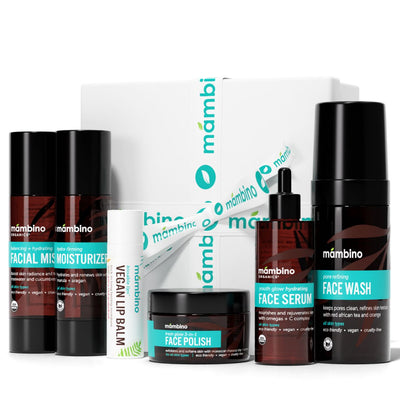The image showcases a comprehensive face care pack by the brand Mambino, presented as an appealing product advertisement. Centrally featured is a white gift box adorned with a white and blue ribbon, with "Mambino" inscribed in multiple ways. The set includes a variety of skincare products, all housed in distinctive brown and black bottles with teal blue labels. From left to right, the collection contains two tall bottles of facial moisturizer, a white tube of vegan lip balm, a smaller container of face polish, a medium-sized bottle of face serum, and the largest bottle labeled face wash. The overall presentation suggests that the products are suitable for all genders and are neatly arranged to highlight the elegant branding and cohesive design of the Mambino face care line.